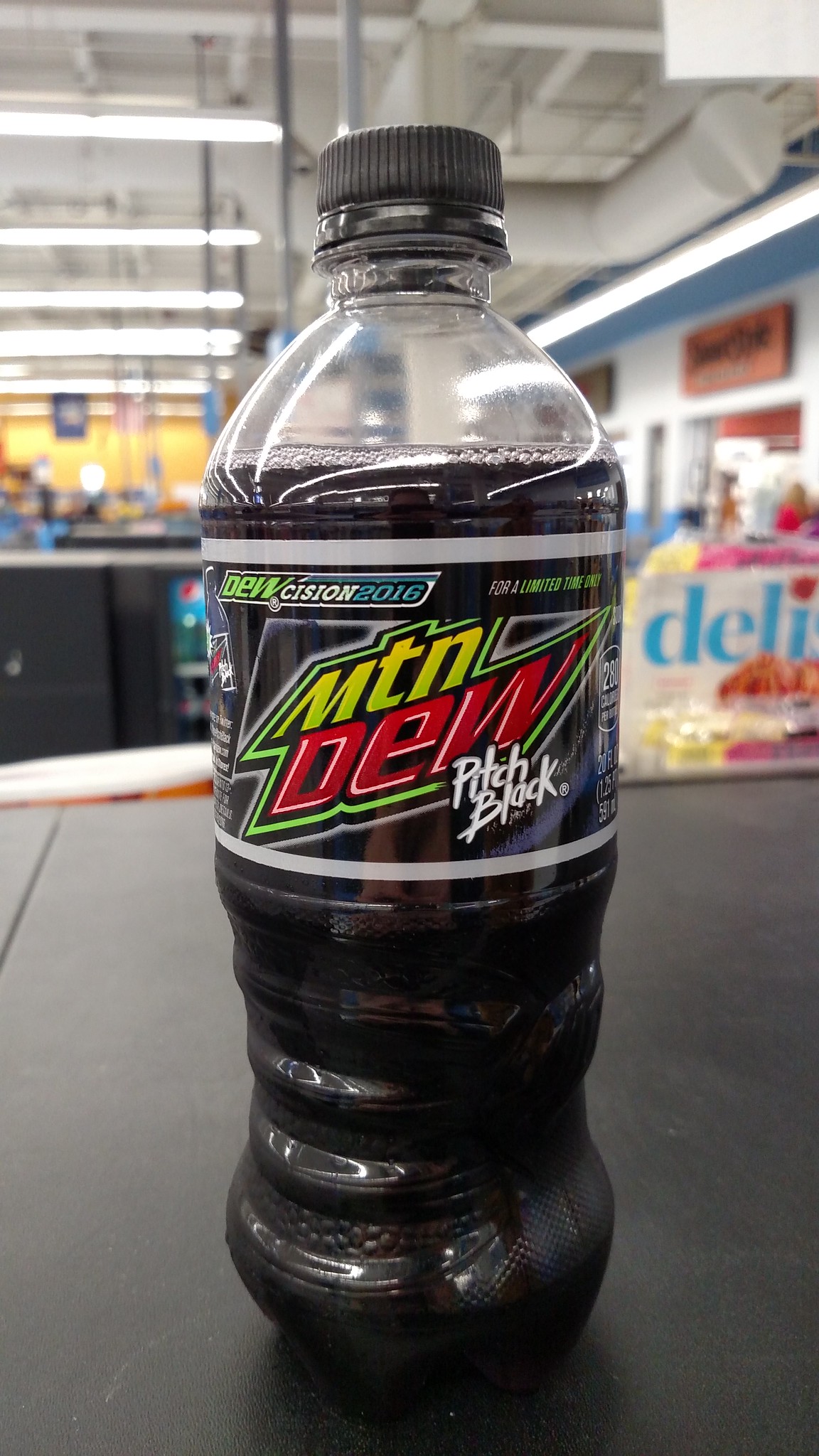In this image taken inside a store, a Mountain Dew Pitch Black beverage is being purchased and is positioned on a familiar-looking conveyor belt at the checkout counter. The Mountain Dew label is prominently visible, with the drink's signature branding displayed in green and red hues. The words "MTN DEW" are clearly printed on the front. Below this, "Pitch Black" is inscribed in white text, likely indicating a special edition from 2016. The label also mentions "For a Limited Time" and denotes the caloric content, which appears to be something in the 280-calorie range. The liquid inside the bottle is dark, matching the "Pitch Black" theme, and the bottle cap is black as well.

The surroundings of the image reveal a black countertop, contributing to a cohesive aesthetic with the dark-themed soda bottle. On the middle right, there is a partial label that reads "Delish" or something similar, suggesting a promotional ad or product name nearby. The right side of the image features a plain white wall adorned with a large sign displaying black text, which is not fully legible. Overhead, the ceiling is grey with visible fluorescent lights illuminating the area. In the distant background, a yellow wall and additional store shelving can be seen, indicating this setting is part of a larger shopping center.